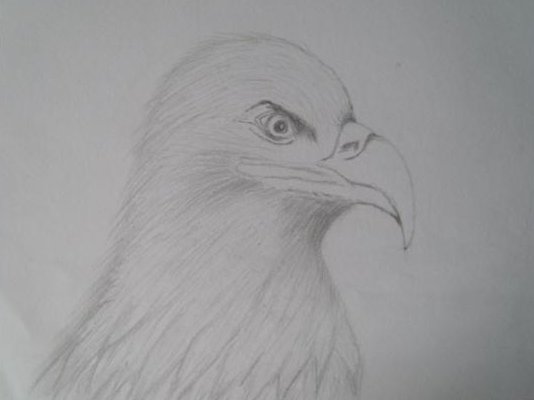On a gray piece of paper, an intricately detailed pencil drawing depicts a fierce bird of prey. The bird's menacing gaze, accentuated by a dark shadow around its eye, exudes a sense of anger and intensity. Its sharp, curved, and somewhat elongated beak adds to its predatory appearance. The bird's head is rounded and predominantly gray, with feathers that vary in shades from light to dark gray, creating a layered effect throughout its plumage. The overall portrayal highlights the bird's formidable nature, especially emphasized by its piercing, almost sinister eye.